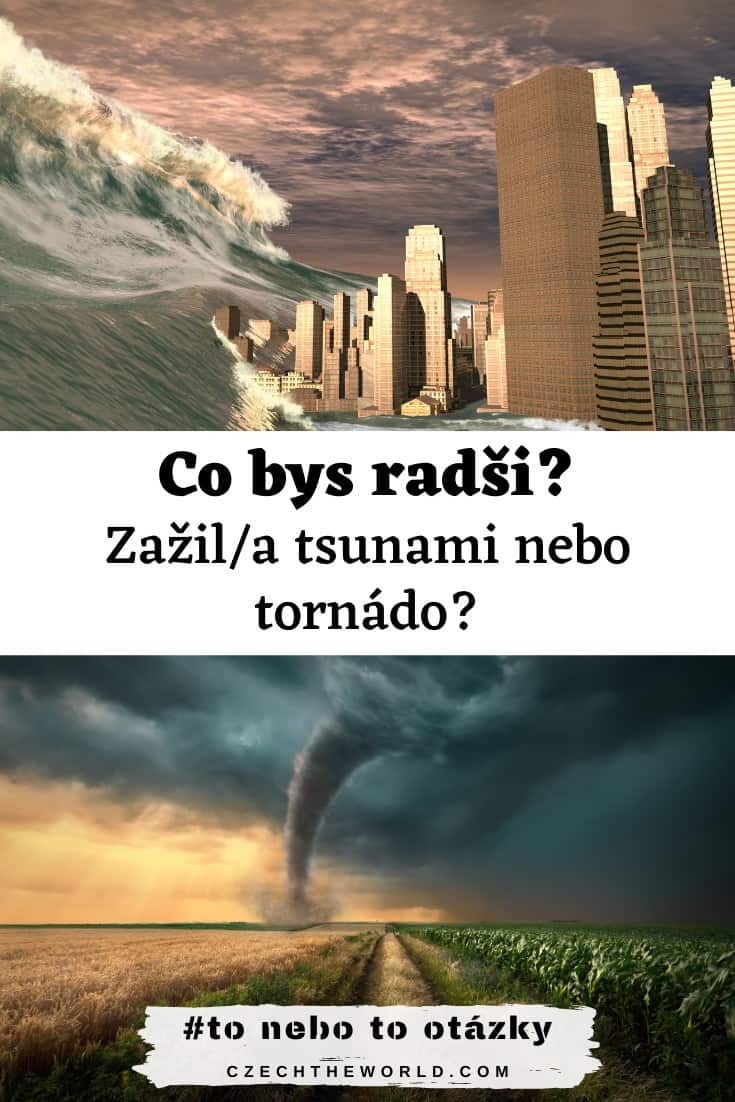This image, possibly a poster from the Czech Republic, depicts two simulated natural disasters with vivid detail. The top half shows a colossal tsunami advancing from the left towards a large city with tan-brown skyscrapers. The sky is rendered in ominous shades of purple and gray, suggesting an impending catastrophe. Inscriptions in Czech, including "Kobis Red Sea?" and "Zasila Tsunami Nebo Tornado?" alongside question marks, indicate a sense of inquiry or speculation about the disaster. The bottom half of the image portrays a fierce tornado twisting through a crop field, juxtaposed against a background where the sun appears on the left and dark, stormy clouds dominate the right. At the very bottom of this section, more Czech text reads "Tu Nebo To Otazki," alongside the phrase "checktheworld.com," with "CZECH" emphasizing its connection to the Czech Republic.